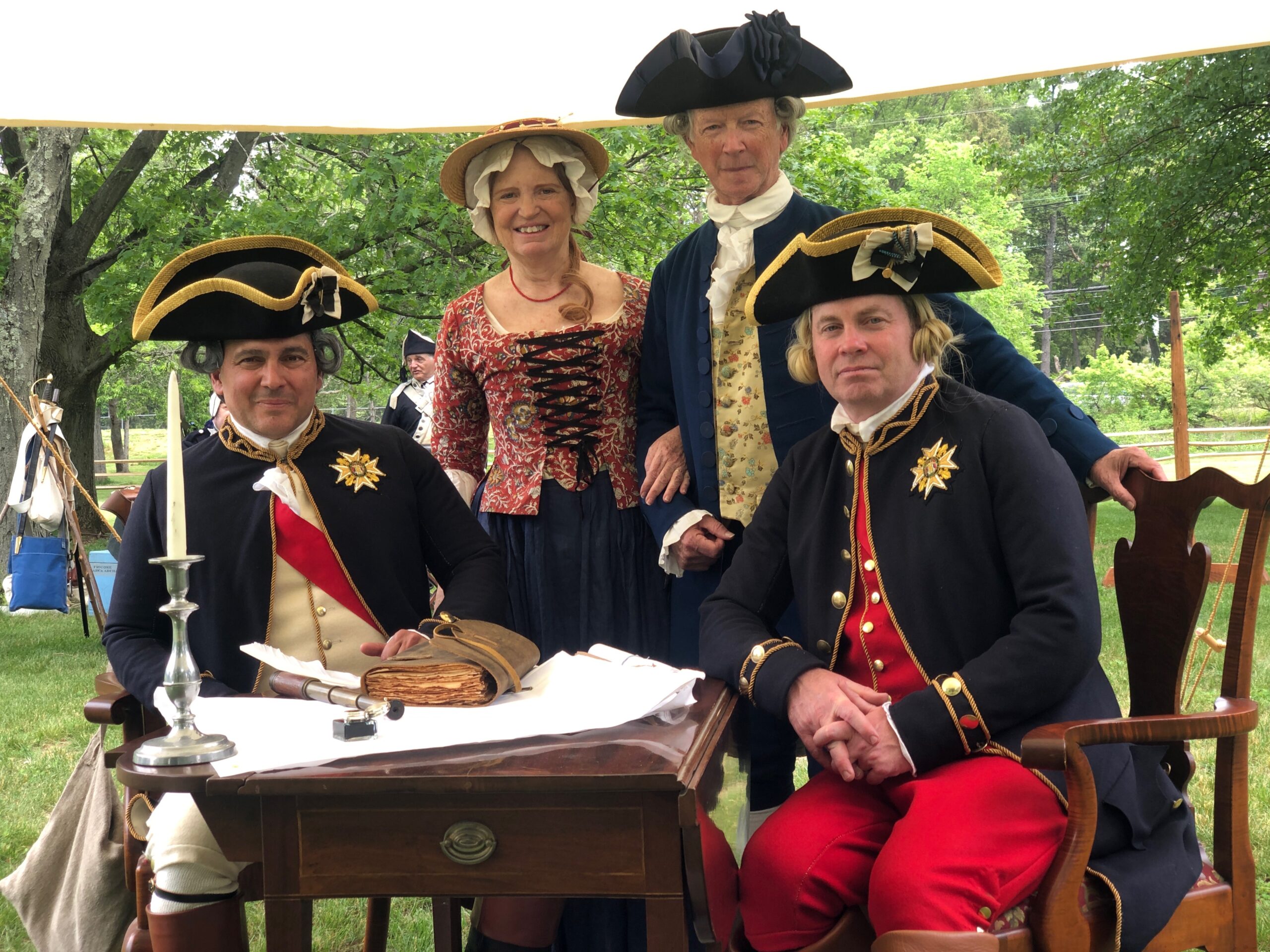The image showcases a detailed and vibrant reenactment of the Revolutionary War, featuring four individuals adorned in authentic period attire. On the left, a man in a tricornered black hat with a gold rim sits behind a rustic brown wooden table. He has a curled wig of black and white hair and is dressed in a distinguished blue jacket with a gold military star, accented by a white undercoat and a striking red sash. His white knickers and brown boots complete the look. Before him lies a brown leather-bound book with old-style papers, an ink bottle beside a scroll, and a quill pen poised in his hand. The table also holds a silver candlestick with a white candle.

Beside him stands a woman with white skin and red hair, her ensemble including a red corset, a blue skirt, and a straw hat with a linen cover draping over her head. Her arm links with that of an older man, who sports a white and gray curled wig topped by a black military-style hat. He is dressed in a blue jacket and matching blue knickers, adorned with white socks. 

To the right is another seated man in a black military hat with gold fringe, wearing a blonde curled wig and similar military attire - a dark ornate coat with gold bands on the collar and cuffs, a red vest, and red knickers, paired with brown boots. The scene is set outdoors on a sunny day, with trees faintly visible in the background. They are all gathered around a small wooden desk that also features a Queen Anne-style mahogany chair, completing the historically rich tableau.